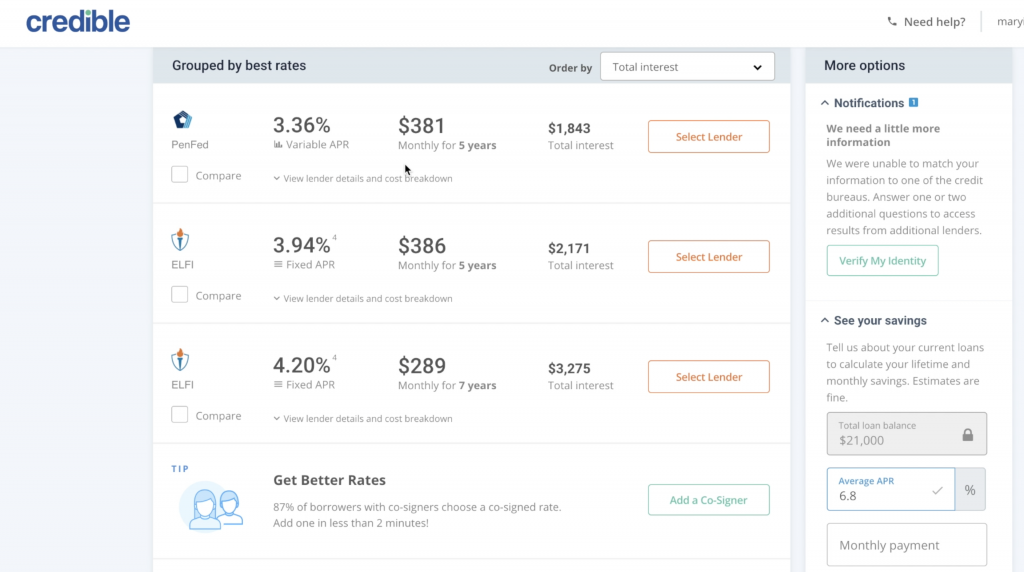Screenshot of Credible Interest Rates Dashboard

The image displays a widescreen screenshot from the Credible platform, typically used for comparing interest rates. The screen is divided mainly into two sections. The prominent left-hand section is titled "Grouped by Best Rates," where a series of interest rates from different providers are listed. Specific providers mentioned include PenFed and ELFI, with varying annual percentage rates (APRs) detailed as follows: 3.36%, 3.94%, and 4.20%. Next to each rate, total interest amounts and a "Select Lender" button are visible, allowing users to choose their preferred loan providers.

On the right side, the second section features additional options such as information about notifications, savings, total loan balance, average APR, and monthly payment boxes. A drop-down menu is available for selecting different criteria or options, and "Order by Total Interest" is another sorting option presented in this section. The layout and information suggest a comprehensive tool for users to compare loan rates and financial details effectively.